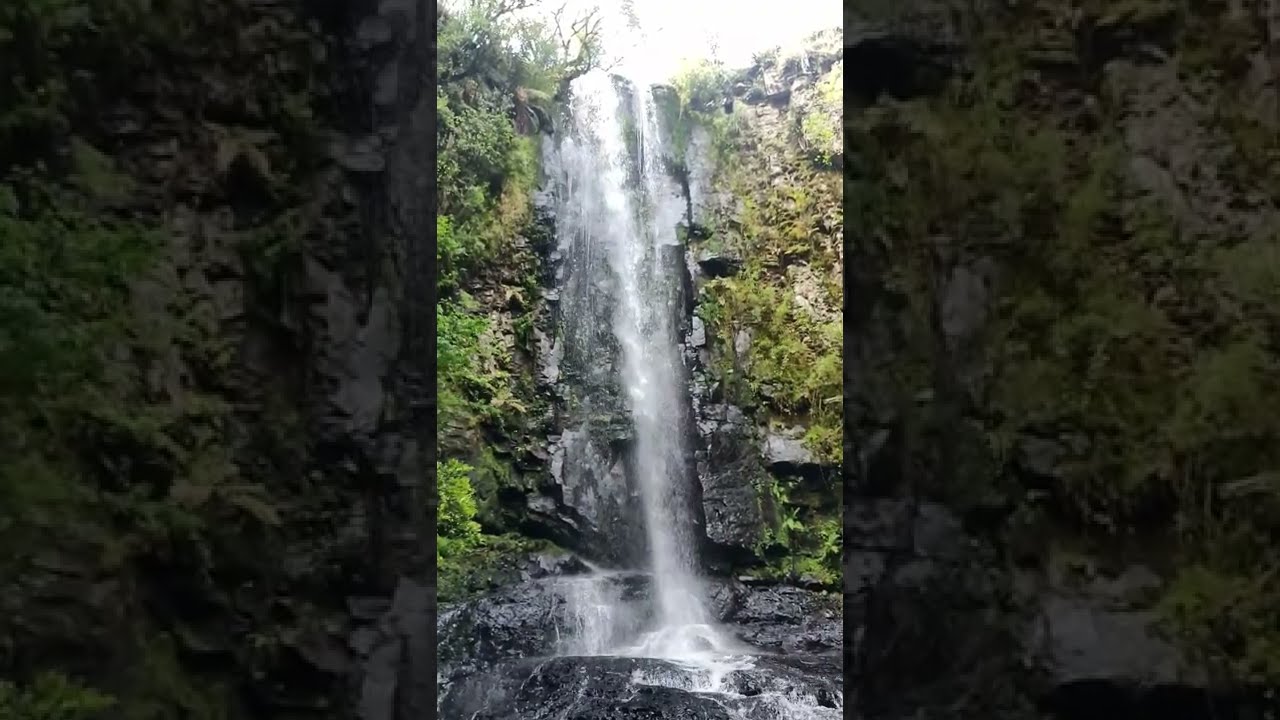The photograph captures a striking vertical composition of a waterfall descending from a high, rocky cliff into a turbulent stream below. Dominating the center of the image, the narrow waterfall cascades down a 30-foot drop, crashing onto an array of slick, dark rocks rather than forming a pool. Flanking the central cascade, two rectangular insets show zoomed-in sections of the same waterfall, highlighting its detailed texture and force. The cliff is a rugged rock formation with a rich brown hue, adorned with lush green vegetation, including moss, plants, and tall green trees whose branches stretch out, enhancing the vibrant, natural setting. The sky peeking through above is bright and clear, indicating a non-overcast day. The sheer rock face appears soaked and slippery, giving a sense of the waterfall's powerful flow and the wild stream it feeds into. Taken with a smartphone in a vertical orientation, the image presents a dramatic, close-up view of the natural wonder, accentuated by the repeated, magnified sections on either side.